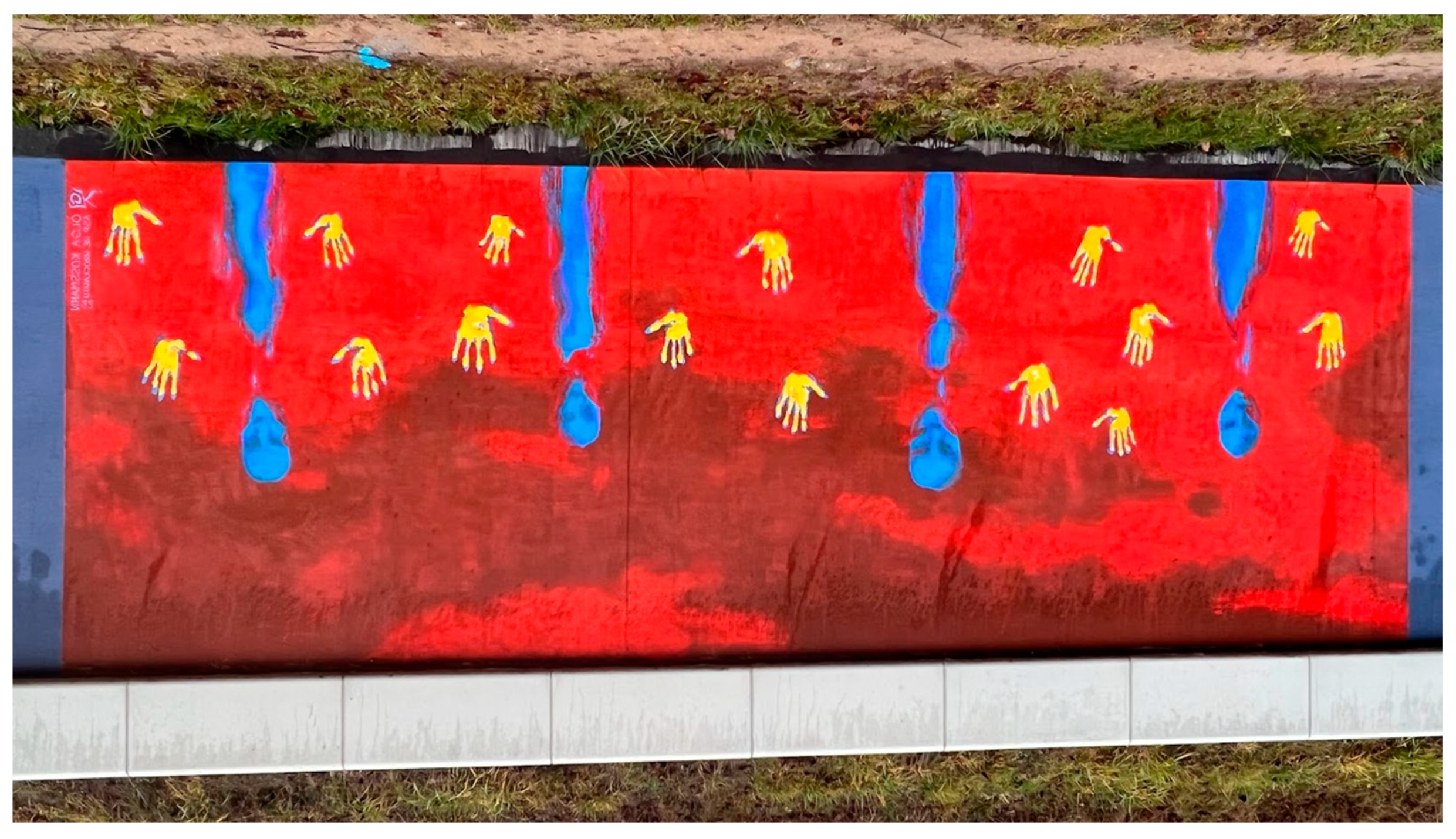The photograph depicts a vibrant piece of artwork on a wall, which initially appears upside down. Dominating the image is a red background, accented with dark red splatters toward what seems to be the top. Yellow human handprints pepper the bottom half of the mural, totaling around fifteen scattered prints. Central to these prints are four blue human-like figures with detailed faces, including eyes and noses, which some described as resembling alien heads. The wall itself is framed by a white blocky border at the bottom, marred with grey splatters, and blue square borders on the sides, darkened by additional blue splashes at their lower sections. Above the wall, in the background, there is a grassy field adjacent to a weathered dirt road, suggesting the photo was taken outdoors. The artwork concludes at the top with a cement block area, further emphasizing the outdoor scene.